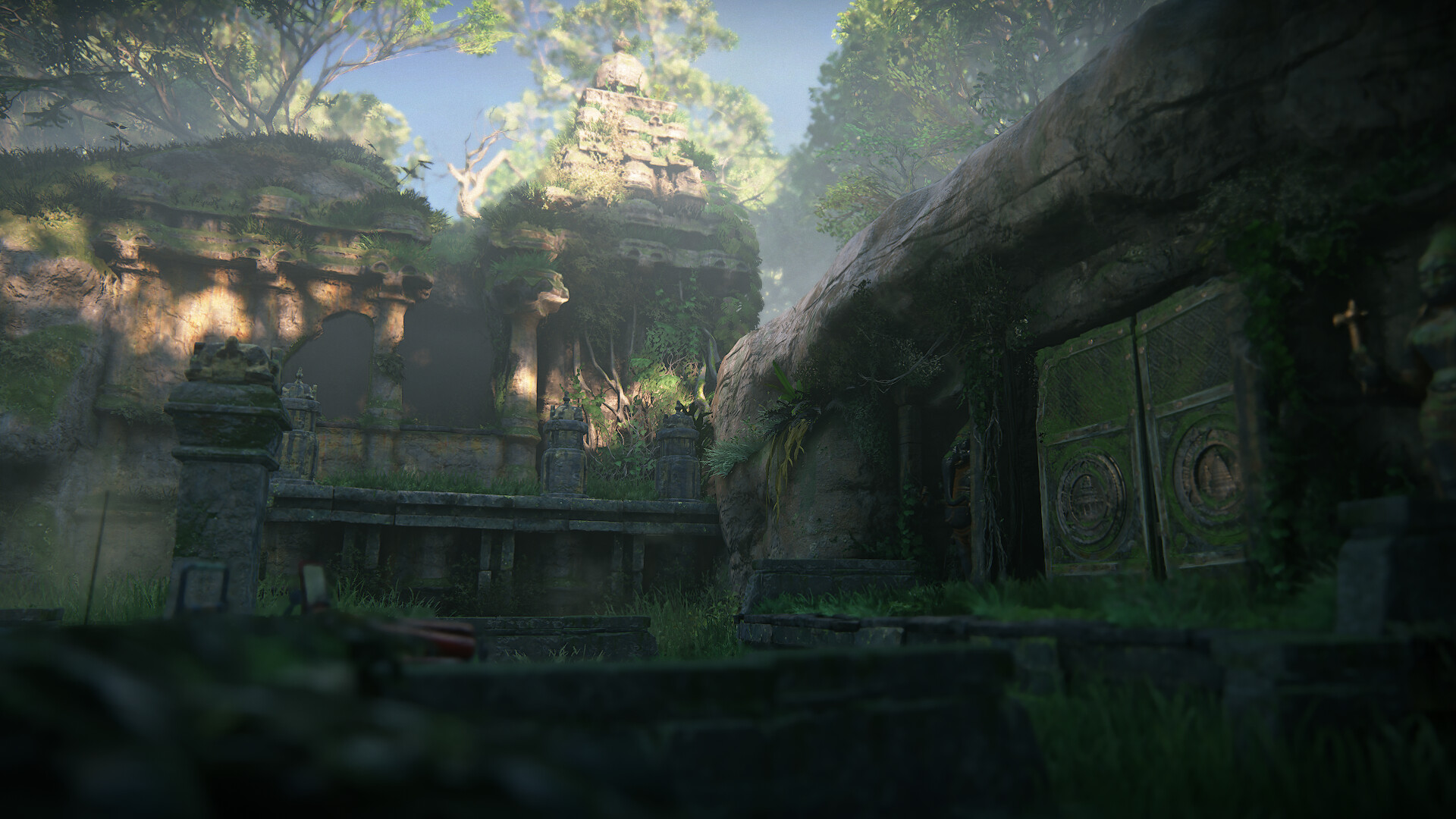The image showcases a detailed video game environment featuring a combination of ancient ruins and natural scenery, captured in a screenshot. Dominated by a bright blue sky, the scene is lit by sunlight that pierces through the otherwise dark setting, casting intricate shadows and illuminating key structures. In the foreground, shadowy buildings, potentially huts or houses, are made of both stone and wood. One prominent structure on the right features two heavy green doors adorned with what seem to be gold or brass accents and large medallion-like circles.

Center to the image is a tall, intricately carved stone temple, distinguished by its pointed peak and perhaps serving as an ancient ruin, hinting at the environment's possibly historical and sacred significance. Beyond the ruins, there is a grassy courtyard area, surrounded by meticulously crafted stonework and garden beds, which blend seamlessly with the grassy mounds and rocks scattered around.

On the right side, a cottage with a stone (possibly thatched) roof and heavy iron doors stands, seemingly built into the side of a mountain. Beside its doorway, a figurine can be spotted. Further in the background, the mansion looms, partially in dappled sunlight, showcasing a second-floor balcony adorned with planters and greenery, supported by an archway with two columns. Tall trees rise behind the mansion, adding to the lush, verdant atmosphere of the scene. This environment, evocative of the video game series 'Uncharted', intricately balances nature and human craftsmanship, combining elements of both stone and organic life.